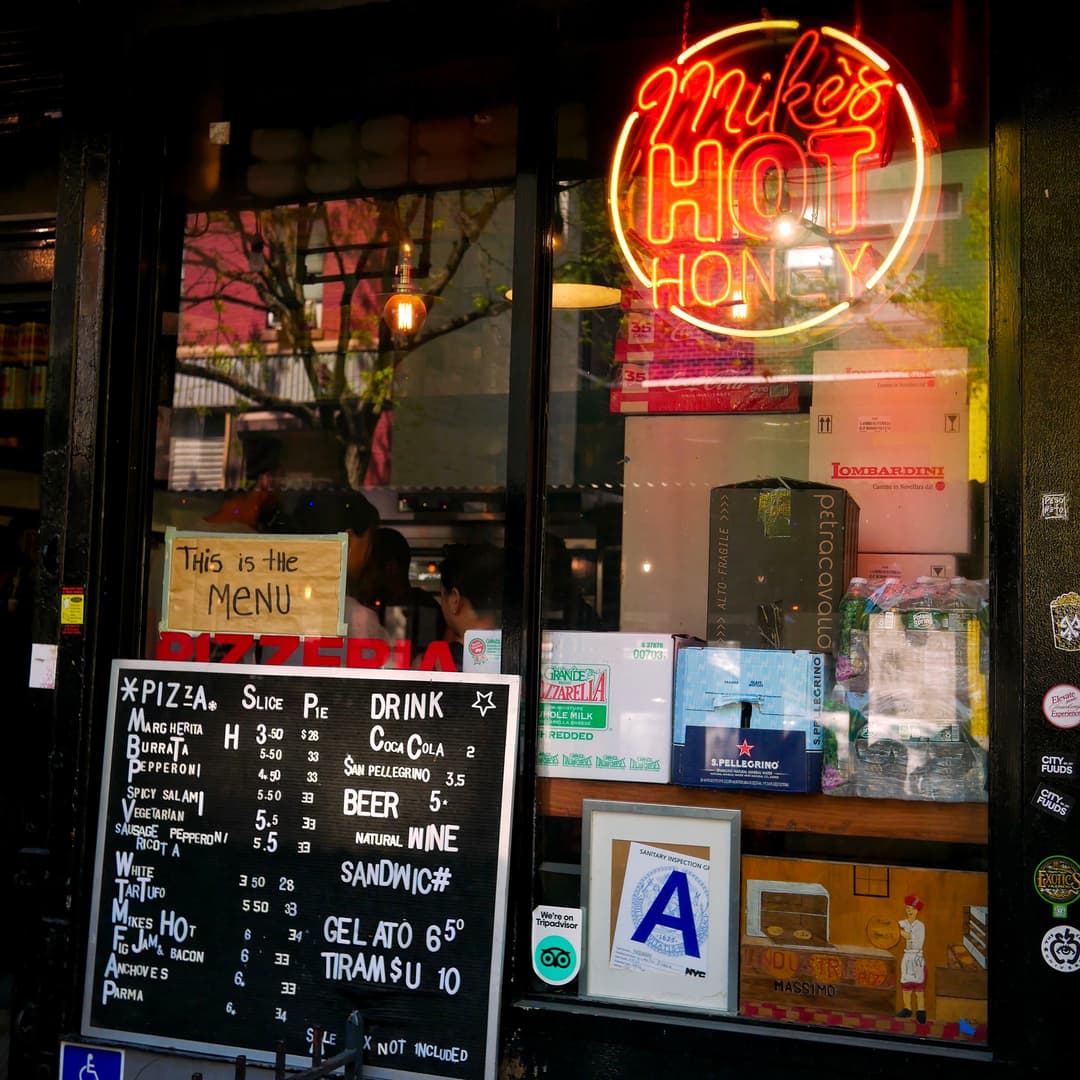The storefront for Mike's Hot Honey is captured in this vibrant photograph. The forefront is dominated by a neon red cursive sign bearing the name "Mike's," with "HOT HONEY" displayed prominently below in all caps. This establishment seems to blend the elements of a pizzeria with a sandwich shop, offering a diverse menu. A black menu board with a white border is visible, showcasing various pizza options such as Margarita ($3.50 per slice, $28 per pie), Burrata ($5.50 per slice, $33 per pie), Pepperoni ($4.50 per slice, $33 per pie), Spicy Salami, Vegetarian, Sausage Pepperoni Ricotta, and White Pizza. Each type of pizza lists prices both per slice and for an entire pie. Beyond pizza, the menu hints at other offerings, including sandwiches, gelato, tiramisu, and an intriguing item called Mike's Hot Fig Jam Bacon. The rustic hand-written menu details, combined with the precise blackboard listings, evoke a cozy yet dynamic culinary experience, potentially located in a bustling neighborhood like Brooklyn, New York.